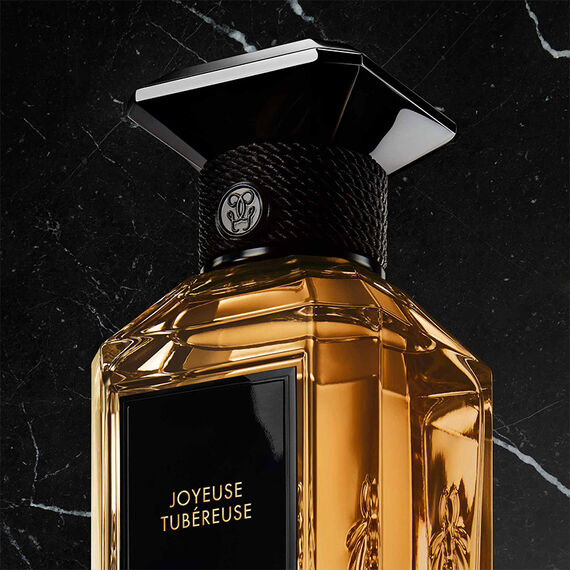This professionally lit advertisement image features a close-up of an angular-shaped glass perfume bottle named "Joyeuse," designed by Toubert Rose. The clear bottle, containing a honey-golden or amber-colored liquid, only partially appears in the frame, focusing on its upper portion. A black, square label with gold, all-caps text on the front prominently displays the perfume's name, "Joyeuse," and the designer's name, "Tuberéuse," underneath. The neck of the bottle is adorned with a small black wax seal featuring a crown stamp detail, which adds an element of luxury. The cap, shiny and black, is shaped like a gem or diamond. The background against which the bottle is set resembles black marble with subtle textural details.